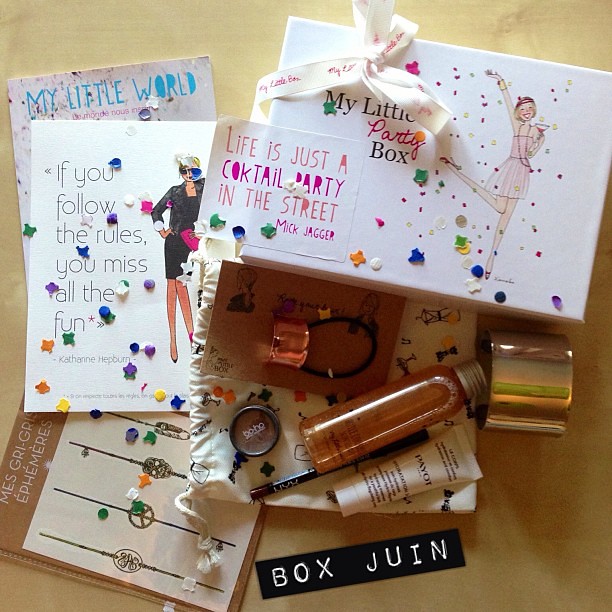The square photograph captures a collection of items arranged on a tan-colored table. Central to the composition is a white box adorned with a ribbon and the label "My Little Party Box." The box features an illustration of a girl holding a martini, with one hand in the air and one leg kicked up. Attached to the box is a quotation by Mick Jagger: "Life is Just a Cocktail Party in the Street." The box is topped with colorful confetti in hues of orange, yellow, green, blue, and purple. To the left of the box lies a series of three papers: the bottom one partially visible with the text "My Little World" in blue, the middle one with a white background displaying a drawing of a woman in a suit jacket and skirt, accompanied by the text "If you follow the rules, you miss all the fun," and the top one featuring a brown frame with images of bracelets, each adorned with charms like a peace sign and a skull. In front of the box is a cluster of makeup items including an orange-colored liquid in a glass bottle, a hair elastic, a tube potentially containing foundation, an eyeliner, and a small circular container possibly holding eyeshadow or blush. To the right of these makeup items is a silver cuff bracelet. Additionally, a white cloth bag with black designs is partially visible, adding to the eclectic assortment of party-themed items.